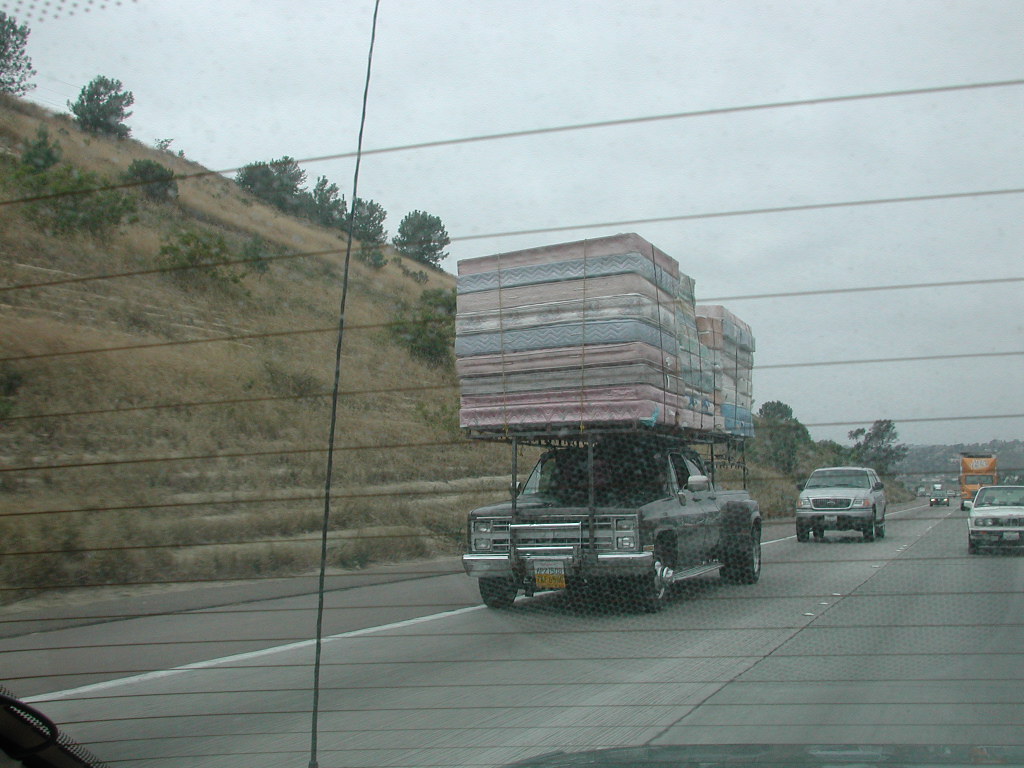The photograph captures a black pickup truck driving down a highway with an extremely precarious load of approximately 10 to 20 mattresses stacked on top. The mattresses are secured on a steel brace with legs that extend down to connect to the truck's front and rear fenders. The truck appears overloaded, with the mattresses towering high above it, posing a significant safety hazard. The scene is viewed through the back window of another vehicle, and behind the laden truck is a gray SUV. To the left of the vehicle, a hill with brown grass and green shrubs is visible. The landscape suggests a southern region, possibly Mexico, California, or Arizona. Additionally, there are four other vehicles in the background, including an orange semi-truck. The overall impression is one of an unsafe and almost comical transportation setup due to the exaggerated load on the relatively small truck.